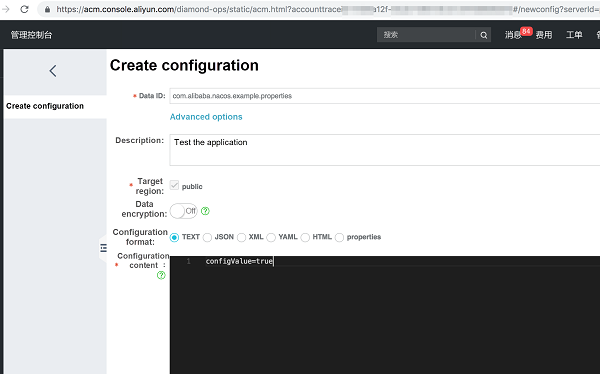Caption:

In this image, a user is configuring settings on a website at the URL https://acm.console.alion.com, with the specific endpoint being partially obscured. The website's interface is primarily black and white, with a few colored elements for emphasis. At the top, there is a search bar containing a partial URL with Asian characters and various parameters such as "accounttrace" and "newconfig?serverid". Below the search bar, the webpage features a thick black header displaying the page title in Asian characters and a numerical indicator '56 or 54' next to another set of Asian characters.

The main section of the page includes a form with fields labeled 'Data ID', which is set to 'com.alibaba.nacos.example.properties', and an 'Advanced Options' section highlighted in blue. The description field reads 'test the application', and the 'Target Region' is set to public, indicated by a checked box.

Data encryption is turned off, with a green question mark icon encircled in green for additional information. The 'Configuration Format' is selected as 'text' via a blue radio button, with other format options including JSON, XML, YAML, HTML, and properties available. The 'Configuration Content' field contains 'config value = true'. Fields marked as required—'Data ID', 'Configuration Content', and 'Target Region'—have red asterisks beside them.